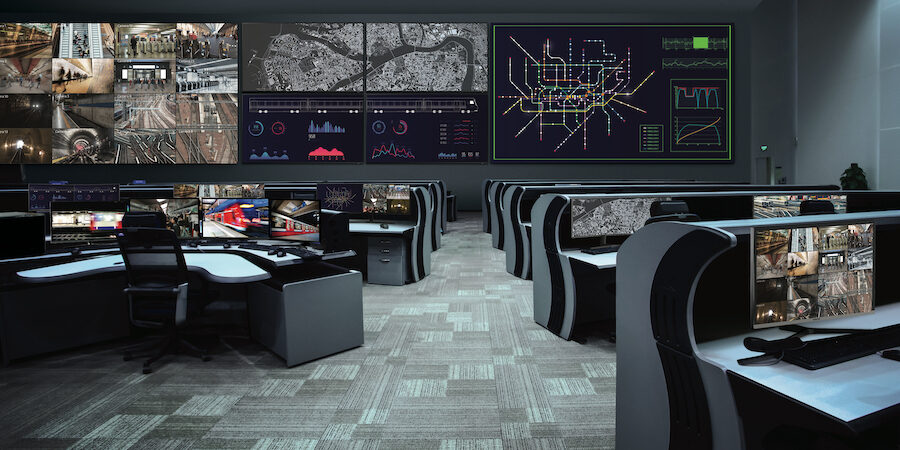The image depicts a large, possibly computer-generated control center interior, reminiscent of a mission control or command room. The space is designed with an open office layout, featuring several desk stations equipped with flat-screen monitors displaying various scenes, including trains. The room is dominated by a bluish-gray color palette, affecting the walls, floors, and desk stations. In the background, a gray wall houses enormous flat-screen monitors, with one prominently displaying a detailed train map. Although the desks are neatly arranged in rows facing the main screens, giving a structured feel to the room, there is no one presently seated at the stations. The monitors on the desks and walls also showcase different images, maps, and charts without any discernible text. The combination of black, red, light blue, yellow, white, gray, dark gray, and green colors adds to the sophisticated and technical atmosphere. Overall, the scene exudes the essence of a high-tech, possibly governmental control center, meticulously equipped but currently unoccupied.